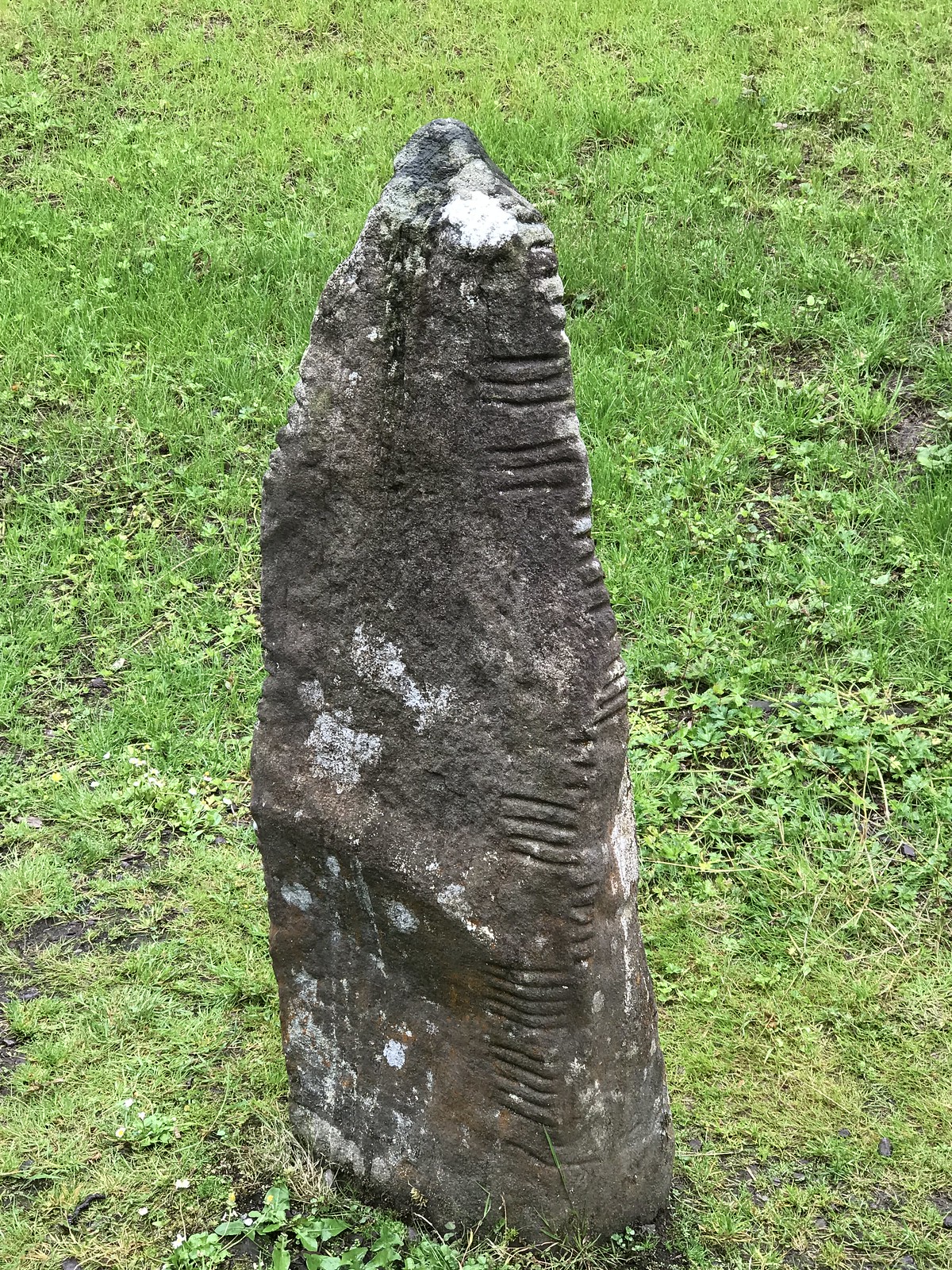The image depicts a tall, irregularly shaped stone resembling a large arrowhead, rising from a vivid, green grassy area interspersed with patches of dark brown dirt. The stone, which occupies the center of the image and extends almost to the top, has a dark gray surface marred by irregular patches of a white, possibly paint-like substance. Towards the right side, ascending the stone, are several groups of horizontal, hand-engraved lines, each cluster comprising four stacked lines that become more densely packed as they approach the sharp, pointed apex. The stone's patina varies from dark, almost black areas to lighter, discolored spots, enhancing its rugged, ancient appearance. This rustic, sculpted stone, with its satisfying, stone-age aesthetic, stands prominently against the lush, vibrant backdrop, creating a striking contrast.